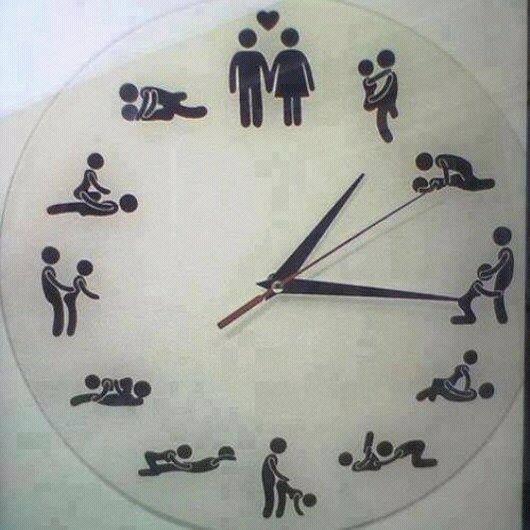This image showcases a unique analog clock with a white face and black hour and minute hands, accompanied by a red second hand. Instead of the traditional numbers, the clock features silhouettes reminiscent of the figures commonly seen on restroom signs, depicting both male and female forms. Each hour position is represented by these figures in a variety of intimate poses, creating a circular pattern of diverse sexual positions. Notably, at the top where the number 12 would typically be, the silhouettes of the two figures are shown holding hands with a heart symbol above them, symbolizing unity and love. The overall background behind the clock is solid white, emphasizing the distinct and unconventional design of the clock face.